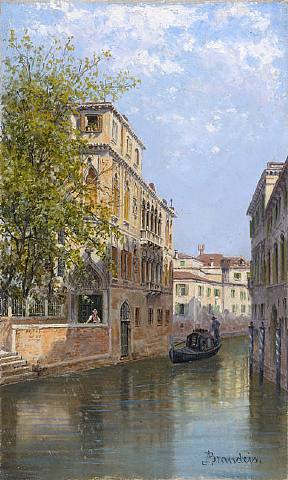The image is an impressionist-style painting depicting a serene Venetian canal nestled between two buildings. The calm, green waters of the canal reflect shadows cast down by the bordering structures. A brown canoe is positioned in the center of the waterway, slightly tilted to the right, with a person dressed in blue standing at the back, appearing to navigate the boat. On the right side, the buildings are predominantly three stories tall, extending to four stories further down. These buildings feature a mix of brick on the lower levels and plaster on the upper segments, with three barber poles affixed to one facade. The building on the left is slightly taller, adorned with a lush green tree in front, whose thick center leaves become sparser towards the edges. Under the tree, a person is seen standing by a brick barrier. The canal extends into the distance, where lighter-colored buildings with amber-hued roofs are visible. Above, a mostly blue sky is dotted with scattered white clouds. In the bottom right corner of the painting, the artist's cursive signature, starting with the letter ‘P’, is visible but not entirely legible.